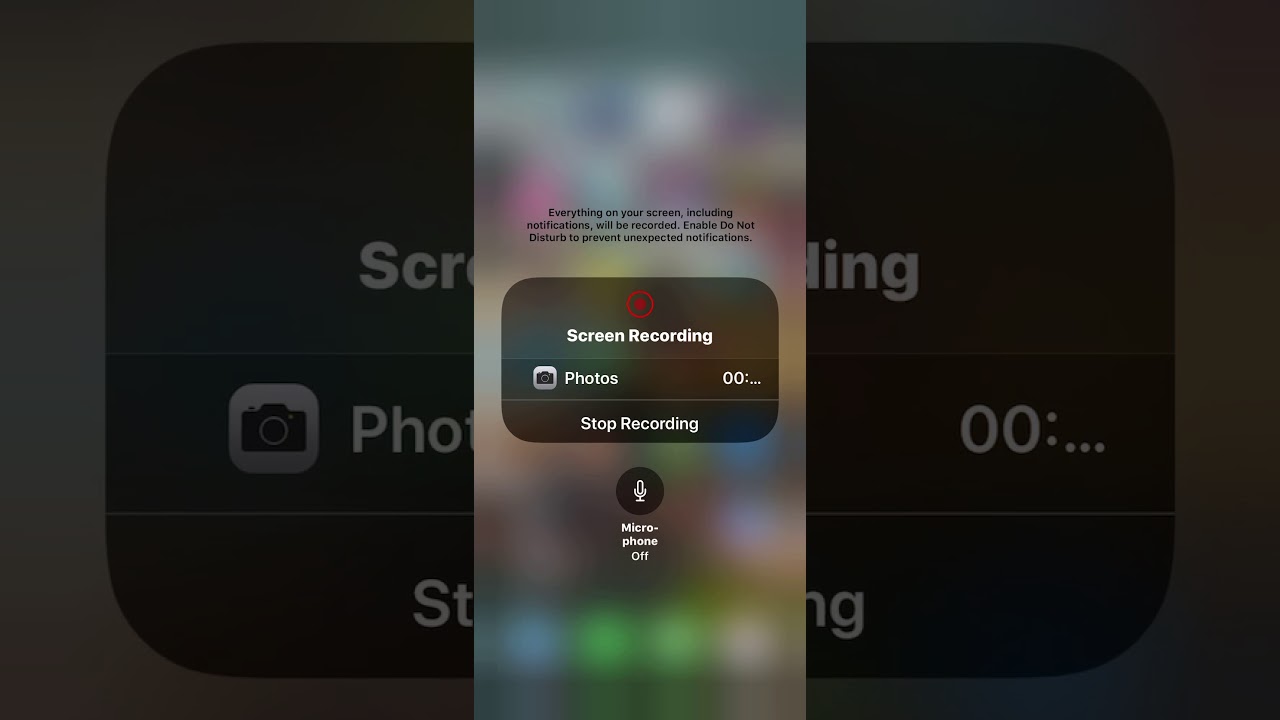The image showcases a device screen recording in progress. Prominently displayed is an overlay message that reads: "Everything on your screen, including notifications, will be recorded. Enable Do Not Disturb to prevent unexpected notifications." The background features a blurred repetition of the same screen, emphasizing the foreground elements. In focus is a black bar displaying text pertinent to the screen recording process and a microphone button. The color palette consists of black, gray, and red, creating a stark contrast that highlights the functional components of the recording interface.